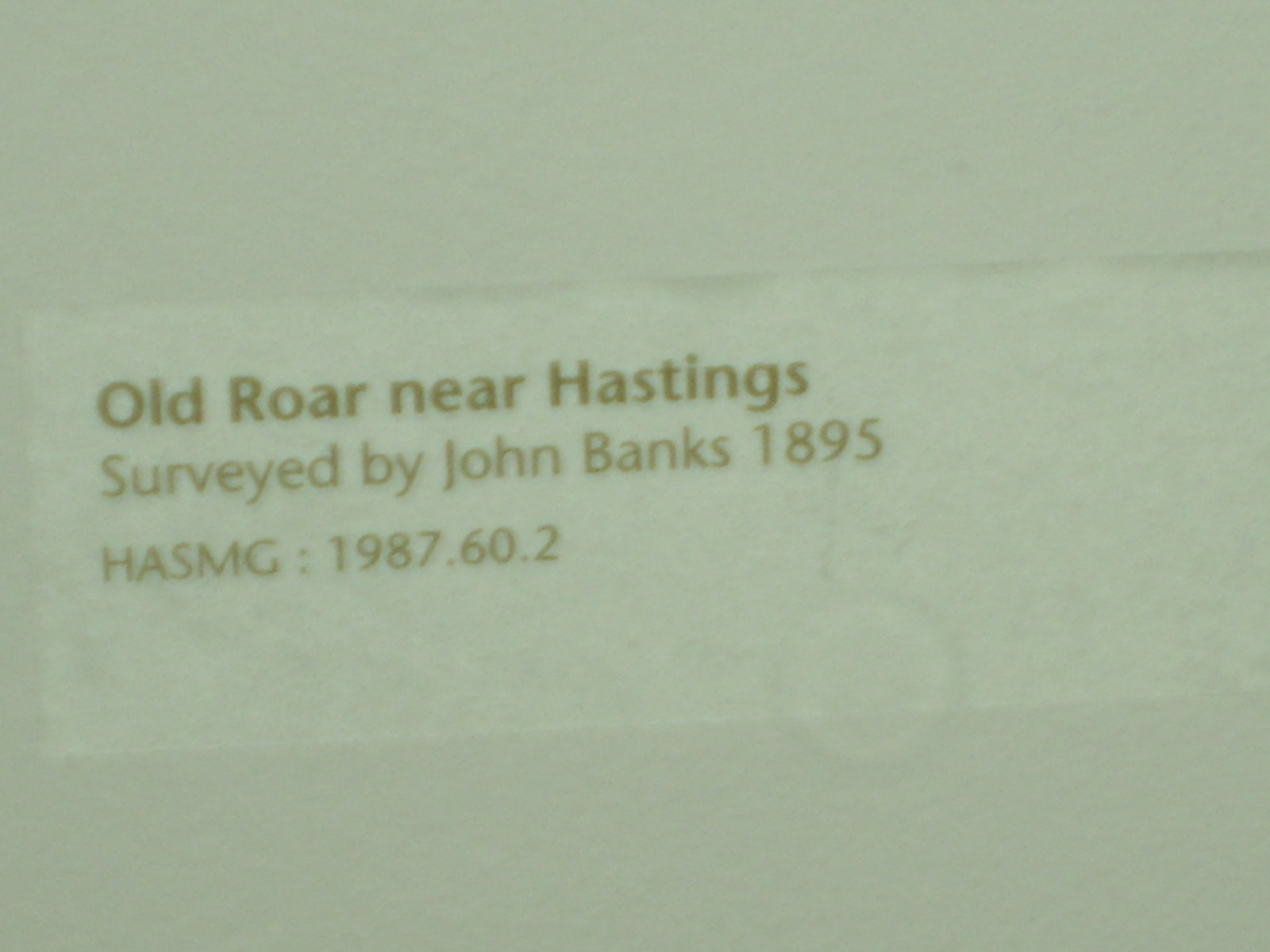The image depicts a faded, rectangular card positioned horizontally with a watermark in the shape of a circle. The card, which has a greenish, off-bluish-white color, features a white band angled approximately 20 degrees from left to right between two darker bands. The print on the card, though somewhat blurry due to image quality, reads "Old Aurora near Hastings" in dark font. Below this, in a lighter font, it states "Surveyed by John Banks, 1895." Following this text, in all caps, is "HASMG: 1987.60.2." The background of the image is plain and empty, accentuating the aged appearance and details of the card.